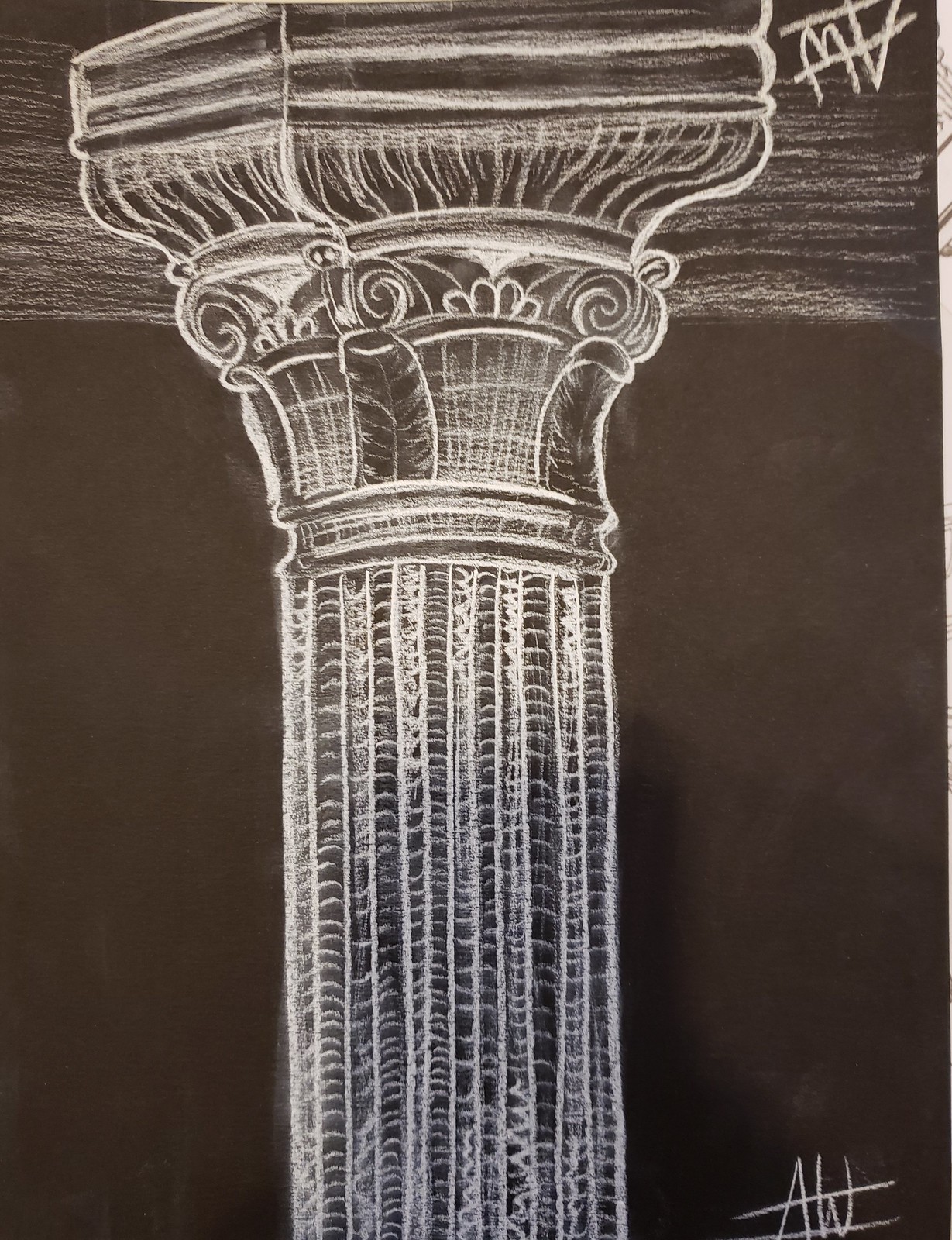This is a meticulously drawn black-and-white illustration of a classical concrete column, reminiscent of those commonly seen in front of federal buildings or courthouses. The column features an intricate lengthwise cutout pattern along its shaft. At the top, it showcases ornate sculptural details, including what appear to be engraved leaves and scrollwork, possibly depicting an acanthus design. The capital of the column broadens slightly, providing sturdy support to the structure above it. The entire scene is set against a solid black background. Notably, there is a signature mark labeled "AW" at the base of the column, with the initials appearing inverted at the top, giving the illusion of "MV."